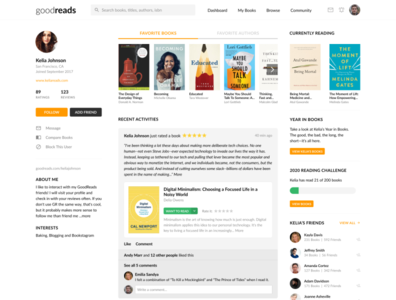A screenshot of the Goodreads website is shown, albeit in a very small and difficult-to-see format. At the top left corner, the Goodreads logo is visible, with 'Good' in light gray and 'reads' in a darker, bolded font. The top menu items are present but not legible due to the tiny size of the screenshot. In the left-hand sidebar is a profile picture of a brunette female, below which are some obscured text likely representing her name, followed by an orange button and a black button, whose functions are unclear. Further down appears a section titled 'About Me,' though it is also hard to decipher. To the right, several icons are shown, representing book covers. Among the seven identifiable icons, the second one seems to be related to Michelle Obama, the third one features a simple pencil illustration, and the fourth has the word 'Talk' with a blue and yellow background. The remaining icons largely lack distinct details, with the third from the end being a noticeable turquoise blue. Below these icons are paragraphs and additional information that remain unreadable in the small-sized screenshot.